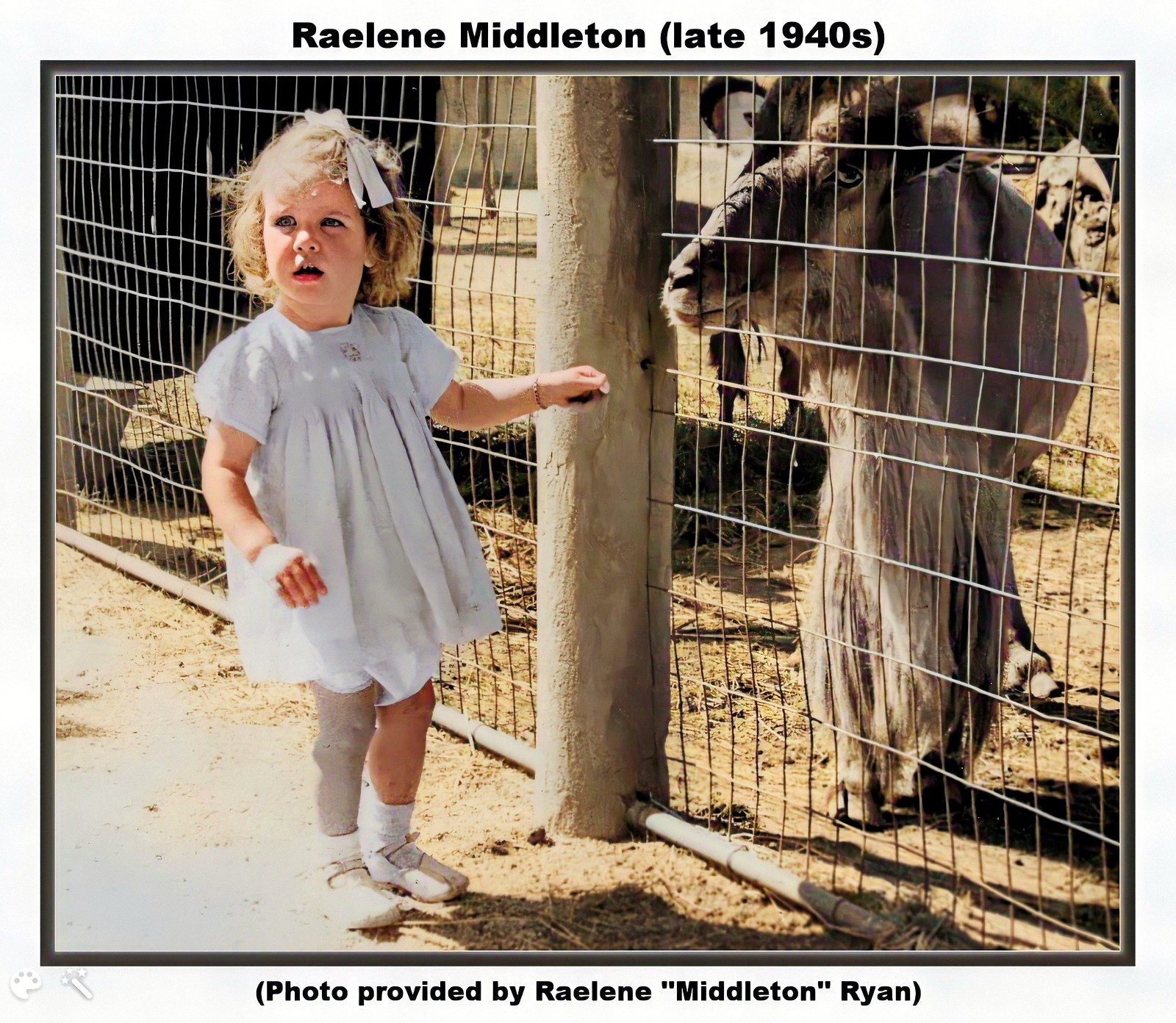The photograph depicts a young Caucasian girl standing in front of a fence, behind which a large brown goat with a long beard and prominent horns peers curiously through the wire mesh. The girl, with shoulder-length curly blonde hair, is adorned with a light baby blue bow and wears a short blue dress reaching her mid-calf, complemented by white socks and ballet-style white slippers. She also sports a bracelet on her left wrist. The scene, potentially set in a zoo or petting zoo, is framed by a solid white border and an inner light gray border, creating a rectangular frame. In the background, the ground is covered with dirt and scattered leaves or hay. At the top of the image, black text reads “Raylene Middleton, late 1940s,” while the bottom caption notes, “photo provided by Raleen Middleton Ryan.”